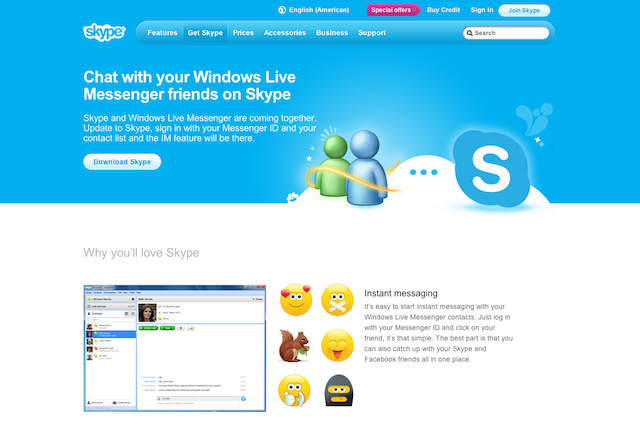This is a vintage screenshot from the Skype website, characterized by its old-style layout and design. The top section features a light blue background, prominently displaying the Skype logo in the top left corner. To the right of the logo is a menu bar with various options: "Features," "Get Skype," "Prices," "Accessories," "Business," and "Support," followed by a search bar.

Above this menu bar is another row containing options such as "English," "Special Offers," "Buy Credit," "Sign In," and a standout button labeled "Join Skype." Below the menu, a prominent white text reads, "Chat with your Windows Live Messenger friends on Skype." Smaller text underneath elaborates: "Skype and Windows Live Messenger are coming together. Update to Skype, sign in with your Messenger ID, and your contact list and the IM feature will be there."

Beneath this message is a white "Download Skype" button. The top section of the page also incorporates graphic design elements, including another Skype logo within the blue background area.

The midsection of the screenshot shifts to a white background, showcasing a banner that reads, "Why you’ll love Skype." Adjacent to this text is a screenshot of the Skype application interface. To the right of the application is a collection of emojis and a paragraph detailing the benefits of Skype's instant messaging feature, completing a comprehensive and nostalgic look at the platform.